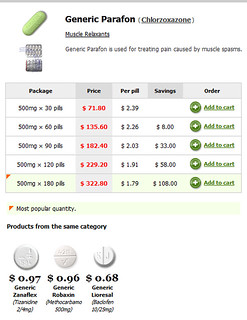Here is a cleaned-up and detailed caption:

---

This image is a screenshot displaying the information and pricing for a generic medication known as Paraffin Chlorzaoxazone, commonly used as a muscle relaxer for treating certain muscle spasms. Prominently featured is an oblong, green pill that appears to be packaged in various quantities, specifically 30, 60, 90, 120, and 180 pills, each with a dosage of 500 milligrams. The corresponding prices for these quantities are listed as $71, $135, $182, $229, and $322, respectively. Additionally, there is a breakdown of the price per pill, noted as $2.39, $2.26, $2.03, $1.91, and $1.79. The screenshot also highlights the savings for customers, with discounts of $8, $33, $58, and $108 for larger quantities. Finally, there is an "Add to Cart" button, indicating that the medication can be purchased directly from the interface.